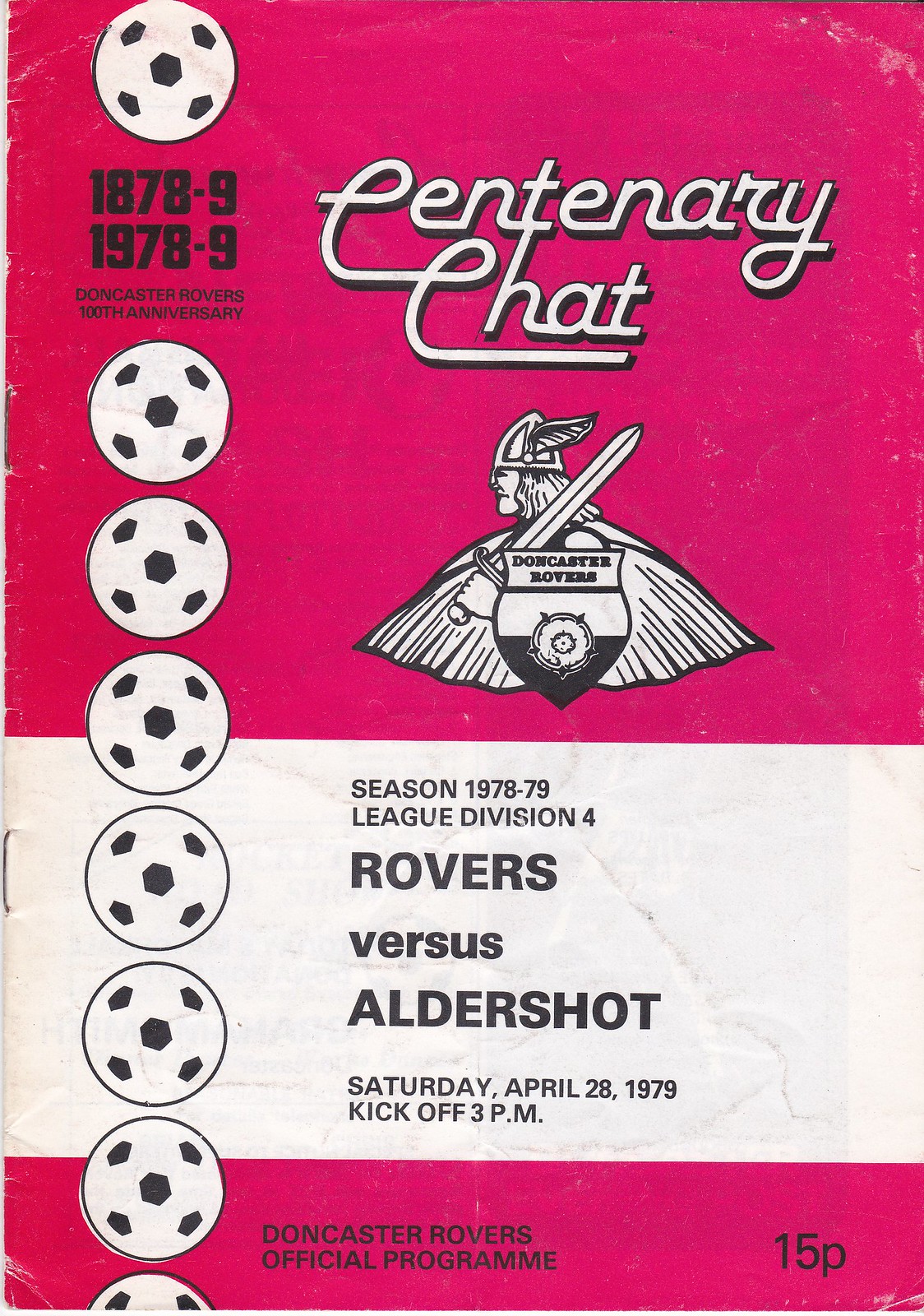The image depicts the front of a matte paper magazine, marked by two visible staples on the left side. The upper half is dominated by a hot pink or reddish color and prominently displays the title "Centenary Chat" in bold white letters. To the right is a vertical column of eight soccer balls. Below the title is a detailed logo of a Viking, shown in profile facing left, holding a large sword on his shoulder, adorned with a cape and a shield.

The text on the cover highlights the Doncaster Rovers' 100th anniversary, with the years "1878-9" and "1978-9" prominently noted. Directly underneath the Viking logo, within a white space, the black text reads: "Season 1978-79, League Division 4, Rovers vs Aldershot, Kickoff April 28th, 1979, Kickoff 3 p.m." At the bottom, in contrasting red and black text, it states: "Doncaster Rovers Official Program, 15p." The overall design and information suggest this was an official match program for a game that took place in 1979.